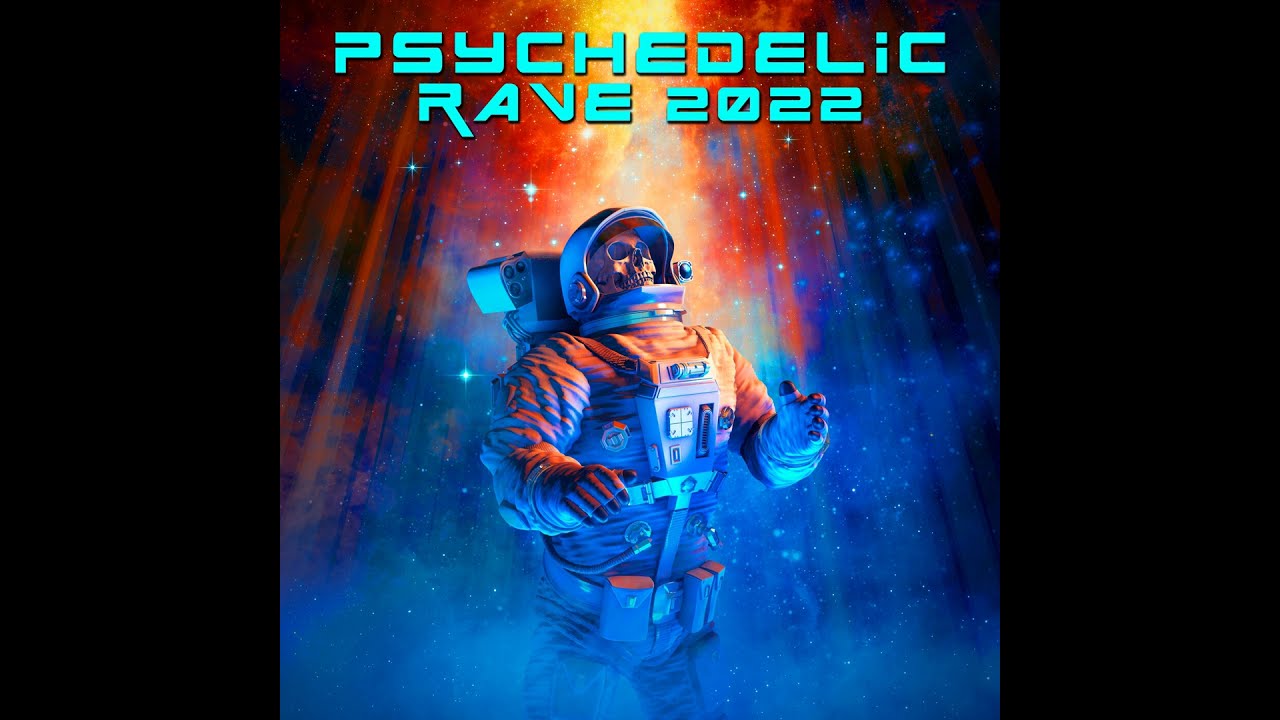This is an artistic and highly detailed poster advertising a "Psychedelic Rave 2022," as indicated by the sci-fi style turquoise text prominently displayed at the top. The central figure is a skeleton dressed in a rust-orange astronaut space suit, complete with a white helmet and utility belt, standing amidst a flurry of stars. The stars near the skeleton's body are blue, contrasting with the bright orange-red star-like beams of light emanating from the top center of the image, which resembles sunlight or a rocket launch. The left and right sides of the poster feature black borders, directing full attention to the captivating skeleton astronaut. The predominantly black, blue, orange, and light aqua color palette enhances the otherworldly, psychedelic theme of the event.